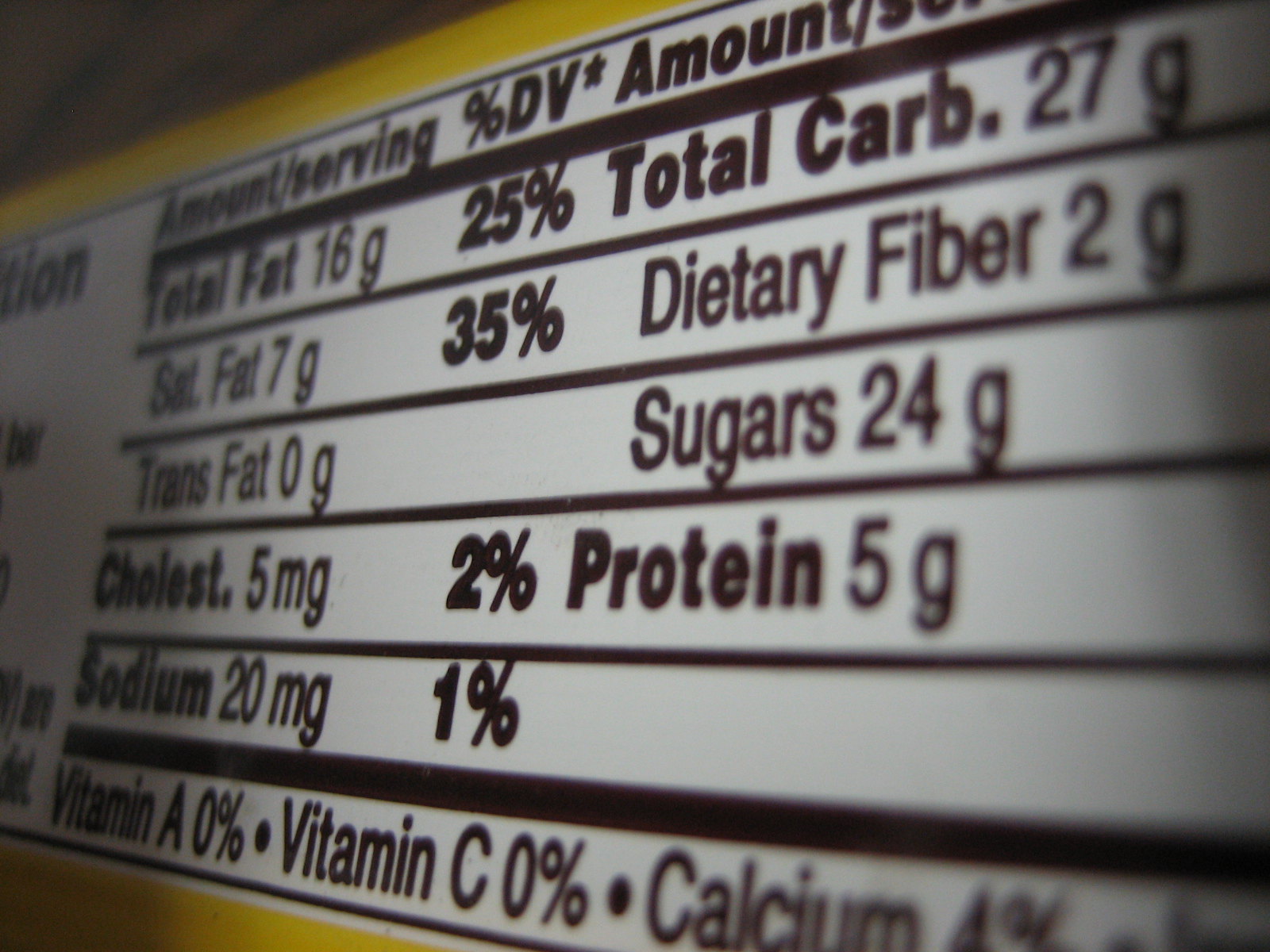This image is a close-up photograph of a nutritional label on the back of a yellow rectangular package of food. The nutritional label itself is white with black font and positioned centrally between the two yellow edges of the package. At the top, it displays "Amount/Serving" and "Percent Daily Values" information. Detailed nutritional facts are listed, including: Total Fat 16 grams (25% DV), Saturated Fat 7 grams (35% DV), Trans Fat 0 grams, Cholesterol 5 milligrams (2% DV), Sodium 20 milligrams (1% DV), Total Carbohydrates 27 grams, Dietary Fiber 2 grams, Sugars 24 grams, and Protein 5 grams. The label also notes that Vitamin A and Vitamin C are 0%, and calcium is partially cut off but appears to be 4%. The photograph captures the label at a slight slant, adding to the close-up effect.